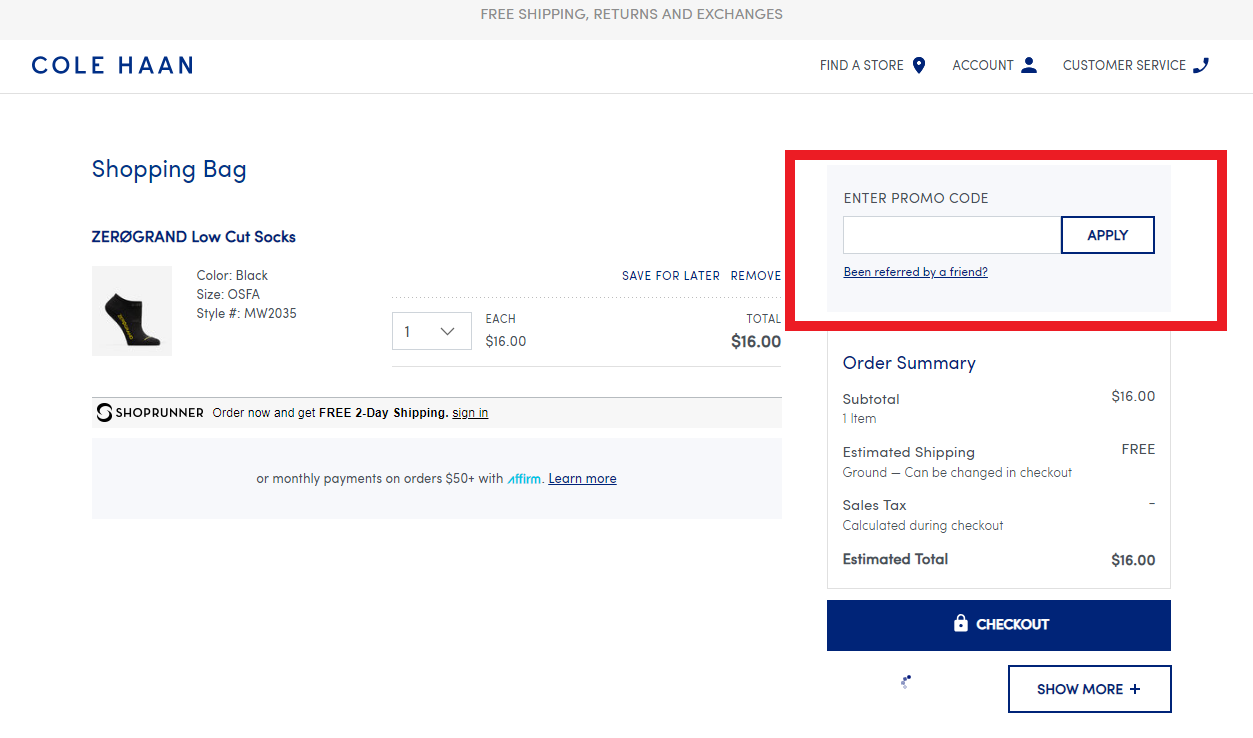This detailed caption provides an intricate description of the elements present on an online shopping checkout page:

"The image displays an online shopping checkout page. Featured prominently at the top are notifications for 'Free Shipping and Returns' and 'Exchanges.' The shopping cart includes a handbag and a pair of black Zero-Gland Low-Cut Socks, listed as style number MW2035, in one-size-fits-all (OSFA), quantity one, priced at $16 each. In the top-right corner of the page, options for 'Find a Store,' 'Accounts,' and 'Customer Service' are visible. A field for entering a promo code is highlighted in red but currently remains empty. The order summary section details a sub-total of $16, with free estimated shipping (with an option to change shipping method during checkout), sales tax to be calculated during checkout, resulting in an estimated total of $16. The colors predominantly used on the page are white and blue."